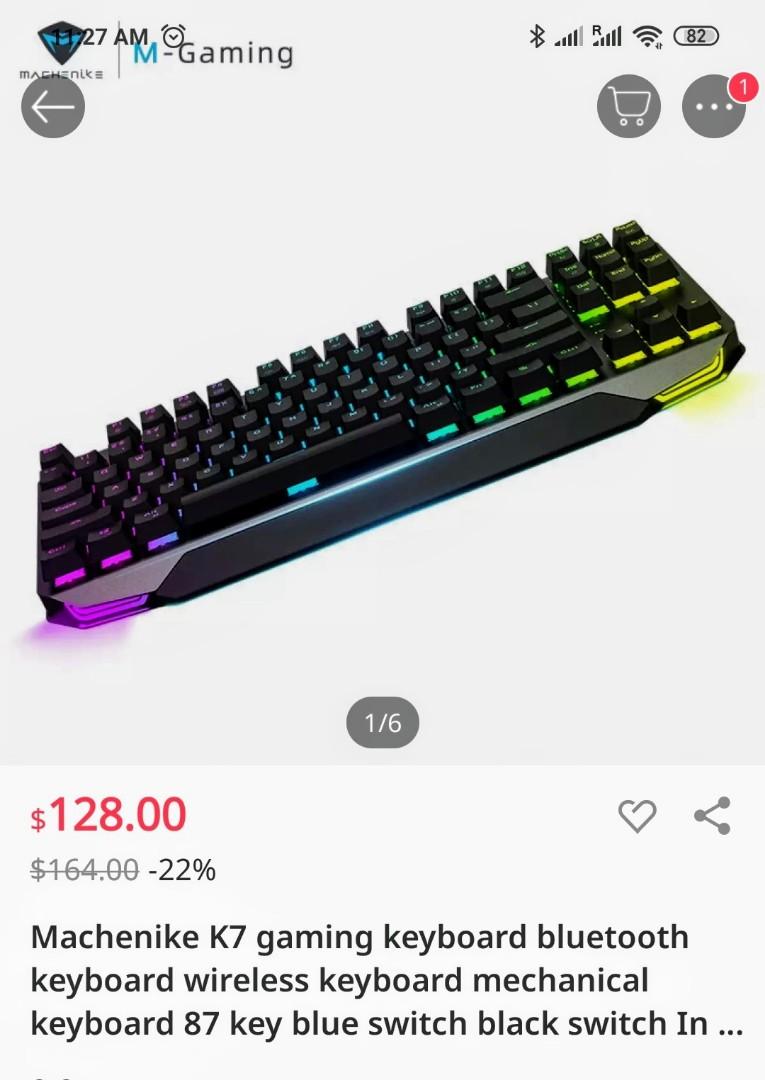In a horizontally rectangular screenshot taken from a cell phone, the top left corner displays the time, partially obscured, showing "XX:27". The top right corner features icons for Bluetooth, signal bars, Wi-Fi, and battery. The main content is an item information page for a keyboard, visible below a back arrow on the upper left, and icons for a shopping cart and a three-dot menu on the upper right. The keyboard image is diagonally positioned from the lower left to the upper right, emanating neon rainbow colors from beneath the keys. Below this image, text reads "Picture 1 of 6". Further down, the item is priced at $128, discounted from $164, indicating a 22% savings. The product is described as the "Mash & Ike K7 Gaming Keyboard," featuring mechanical, wireless, and Bluetooth capabilities, with 87 keys, and options for blue or black switches.